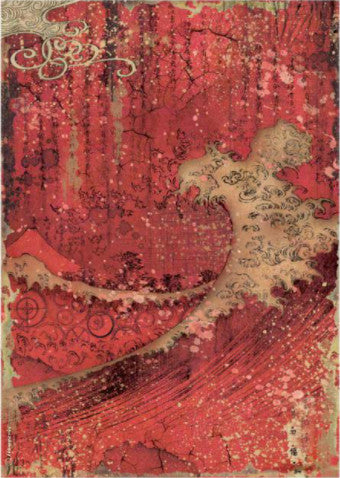This vertical, rectangular image appears to be an abstract artwork featuring a rich tapestry of colors and intricate details. Dominated by various shades of red, the piece also includes striking accents of teal, brown, black, beige, and tan. The central motif involves swirls and waves of these colors, creating a dynamic composition.

The upper left of the image features scroll-like patterns in beige interwoven with black lines, evoking the appearance of tree branches or twigs. Moving towards the center, the red becomes more prominent, shadowed with blacks to suggest ribbed textures or ribbing that runs vertically. This ribbing is intersected by a beige splotch on the middle-right side, which is highlighted with black shading for added depth.

The lower part of the artwork showcases intricate patterns of waves and swirls formed by black lines and bubbles of gray and tan. These elements seem to converge towards the center, giving the piece a harmonious flow despite its visual complexity. Overall, the image is a compelling, busy scene of abstract artistry reminiscent of Japanese rice paper textures, with a strong emphasis on the vivid red hues and detailed black line work that outlines possible natural forms like trees and waves.